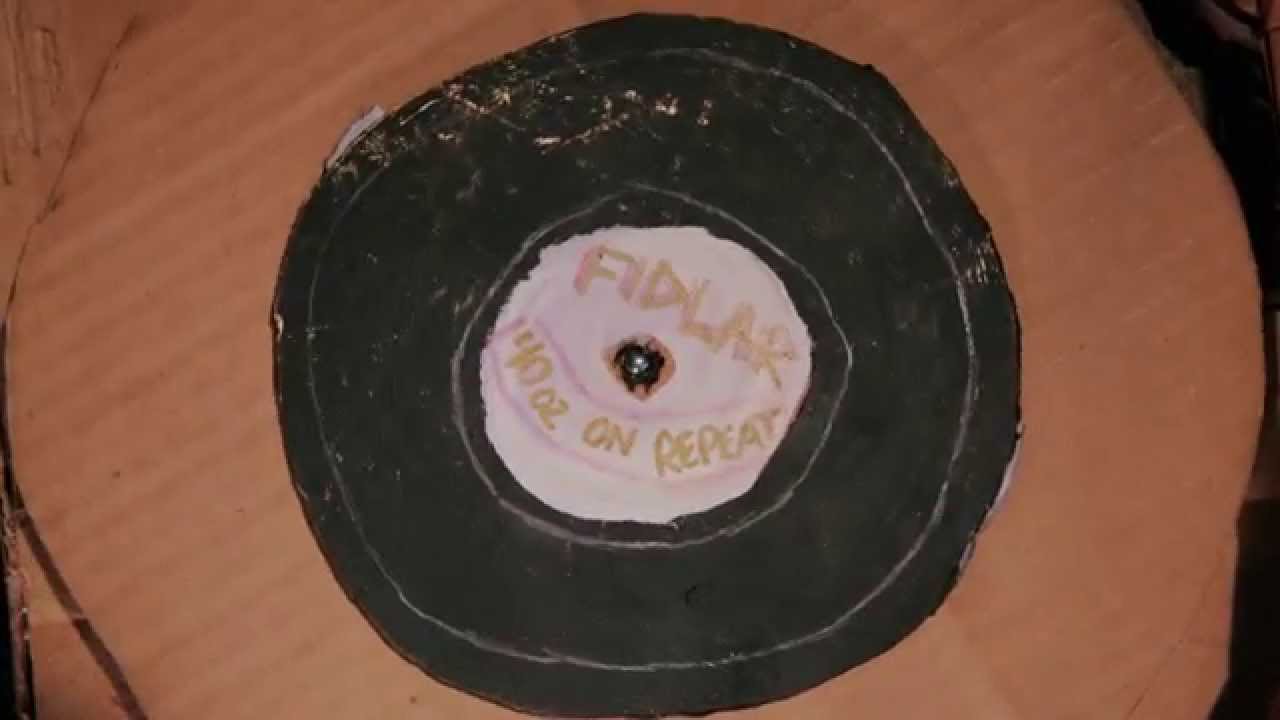The image depicts a handcrafted cardboard representation of a vinyl record. The cardboard is cut into a circular shape, though the top and bottom edges are slightly cropped, indicating it retains its overall circular form. The outer part of the record is the natural brown color of cardboard, while the inner circle is painted black, mimicking the appearance of a classic vinyl record. At the center of the black circle, there's another, smaller white circle, which contains the text "FIDLAR" prominently displayed. Additionally, the text "140OZ" is repeated around this white center. The cardboard has lines drawn on it to replicate the characteristic grooves of a vinyl record, adding to the realistic look of the artifact.